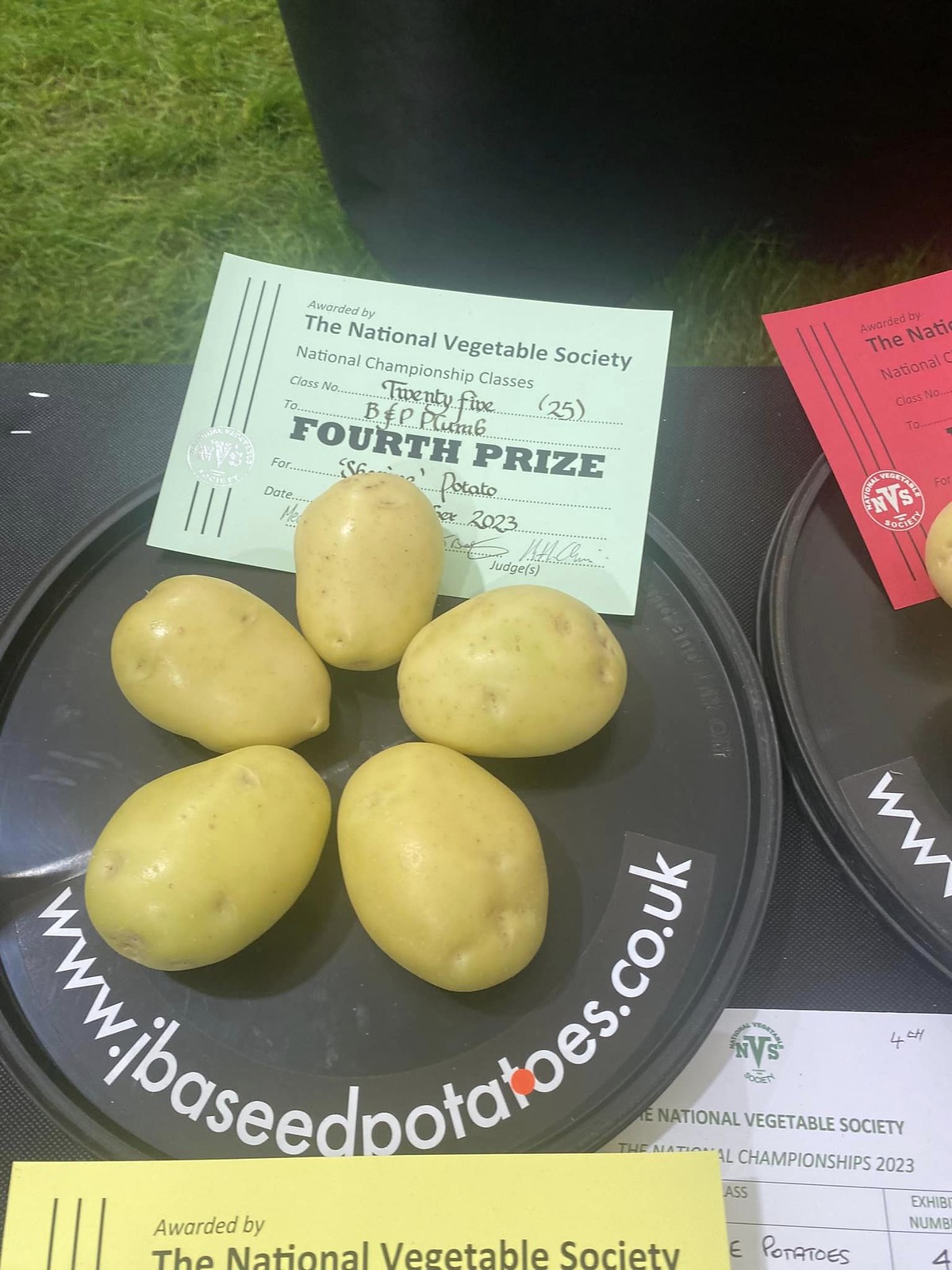This vibrant outdoor photograph, taken at a National Vegetable Society event, showcases a black plate centered on vivid green grass. On the plate, five neatly arranged potatoes earned a commendable fourth prize in a potato contest. The plate prominently displays white, curved text at the bottom, revealing the website "www.jbayseedpotatoes.co.uk". Above the potatoes, a blue rectangular ticket reads "National Vegetable Society, Fourth Prize," likely providing details about the award and the winner. Positioned below the plate is a partially visible yellow card stating "Awarded by the National Vegetable Society." On the far right edge of the image, there's a sliver of another black plate, also inscribed with the same web address, hinting at a larger showcase. The setting—clearly outdoors on grass amidst what appears to be a vibrant vegetable fair or championship—adds to the rustic charm and authenticity of the agricultural celebration.